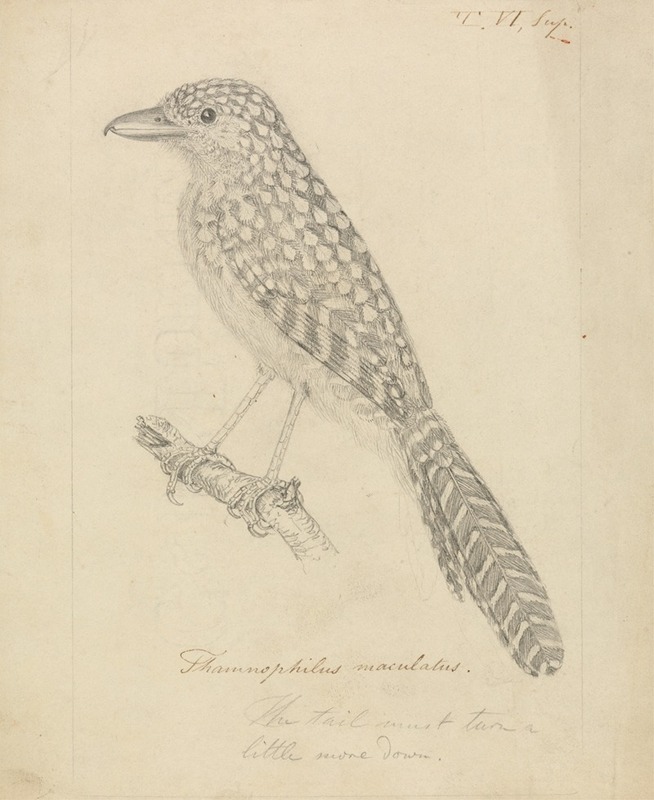The image showcases a vintage-style, black and white pencil drawing of a bird perched on a broken stick or branch. The background is sepia-toned, enhancing the antique appearance, with some cursive inscriptions at the top right, including a Roman numeral VI and the partial word "SUPR." The bird, centrally positioned, is depicted with a long, sharp beak, speckled body adorned with teardrop-shaped white spots, and a tail featuring symmetrical rectangular patterns forming a V shape. Its feet grip the branch, which stretches diagonally from the middle towards the bottom left of the image. At the bottom of the drawing is a handwritten Latin name, "Phamonophilus maculatus," followed by the comment "the tail must turn a little more down," written in cursive.